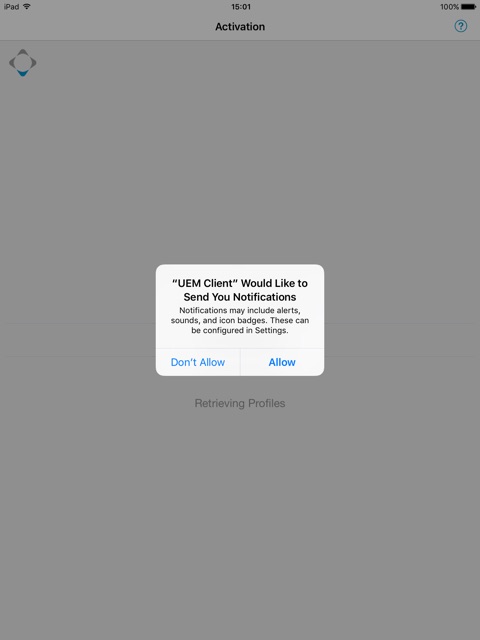A detailed screenshot from an iPad displays an activation page. In the top left corner, the label "iPad" is visible alongside a Wi-Fi icon. Moving to the center portion of the screen, the current time is prominently displayed, while the far-right corner reveals the battery percentage.

Central to the screen, the word "Activation" is clearly positioned with a question mark icon situated to its right. Taking up a substantial portion of the center, a white pop-up box emerges with the message: "UEM client would like to send you notifications" in bold black letters. Beneath this, a smaller line of text informs: "Notifications may include alerts, sounds, and icon badges. These can be configured in Settings."

Towards the bottom of the pop-up box, the options "Don't Allow" and "Allow" are listed in blue text, positioned on the left and right respectively. The underlying screen, largely blank, simply displays the message "Retrieving profiles" in light gray text. 

A distinctive diamond icon with a circle in its center appears in the top right corner of the screen. This icon is primarily purple, featuring a blue point at the bottom of the diamond shape.